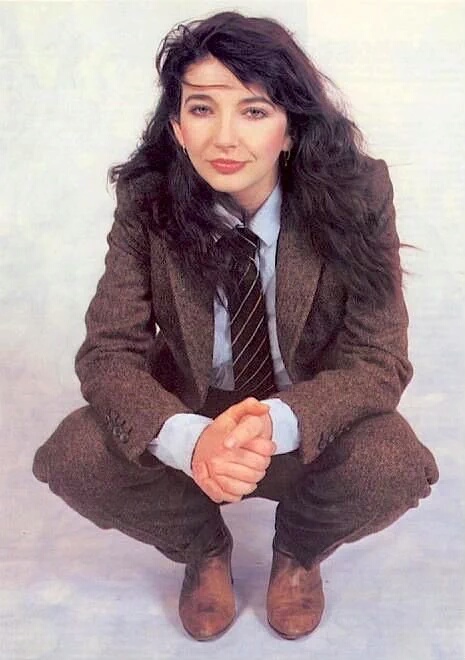The photograph showcases a woman crouching down in a pose reminiscent of a baseball catcher. She is centrally positioned against a grayish-blue background adorned with various spots and shades of white, giving it a cloud-like appearance. The woman has long, wavy, dark hair that cascades below her shoulders and is accessorized with silver hooped earrings. She wears brown pointed leather shoes with zippers on the sides, black tweed pants, and a matching black tweed jacket with three buttoned cuffs. Beneath the jacket, she has on a light blue button-down shirt paired with a black tie featuring thin diagonal silver stripes. Her hands are clasped in front of her, with her elbows resting on her bent knees. She has fair skin, accentuated by red lipstick, and the overall style of the image is a professionally taken portrait.